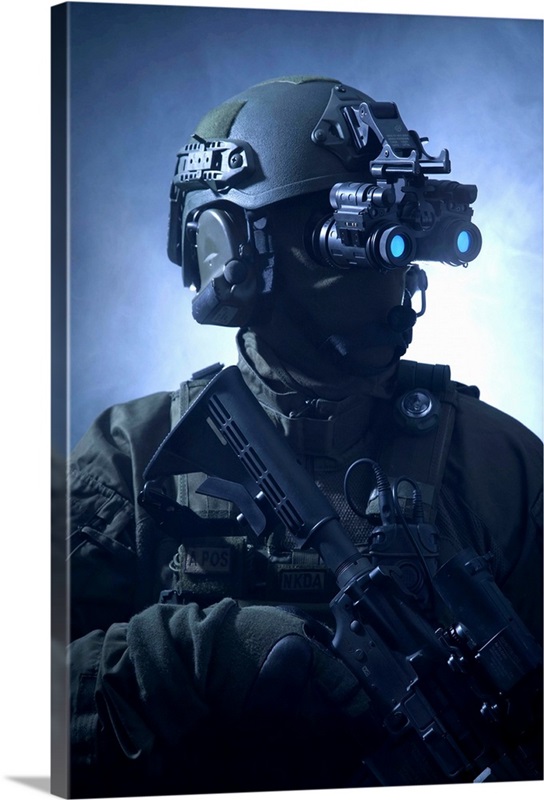The image depicts a detailed and meticulously created digital artwork of a soldier equipped for night operations. The image is presented on a canvas viewed at a three-quarters angle, showcasing both the left edge and the entire front of the piece. Dominated by hues of dark blue, black, and dark green, with a significant portion in shadow, the scene exudes a shadowy, covert atmosphere. The background features a foggy, bluish tone that highlights the soldier's figure.

The soldier stands facing slightly forward and to the right, occupying about 80% of the canvas. He is clad in comprehensive tactical gear, including a dark helmet fitted with night vision goggles that feature striking blue oval lenses, a balaclava that obscures his face, and a suit composed of layered jackets, gloves, and vests. Notably, his vest bears two visible badges: one labeled "A POS" and another marked "NKDA."

He wields an assault rifle, the stock of which is positioned close to his jaw, indicating readiness for action. The distinct mention of no skin being visible reiterates the soldier's complete cover and preparedness for an operation. The dark, shadowy ambiance of the image, along with the soldier's authoritative presence, renders a vivid portrayal of a night ops scenario.